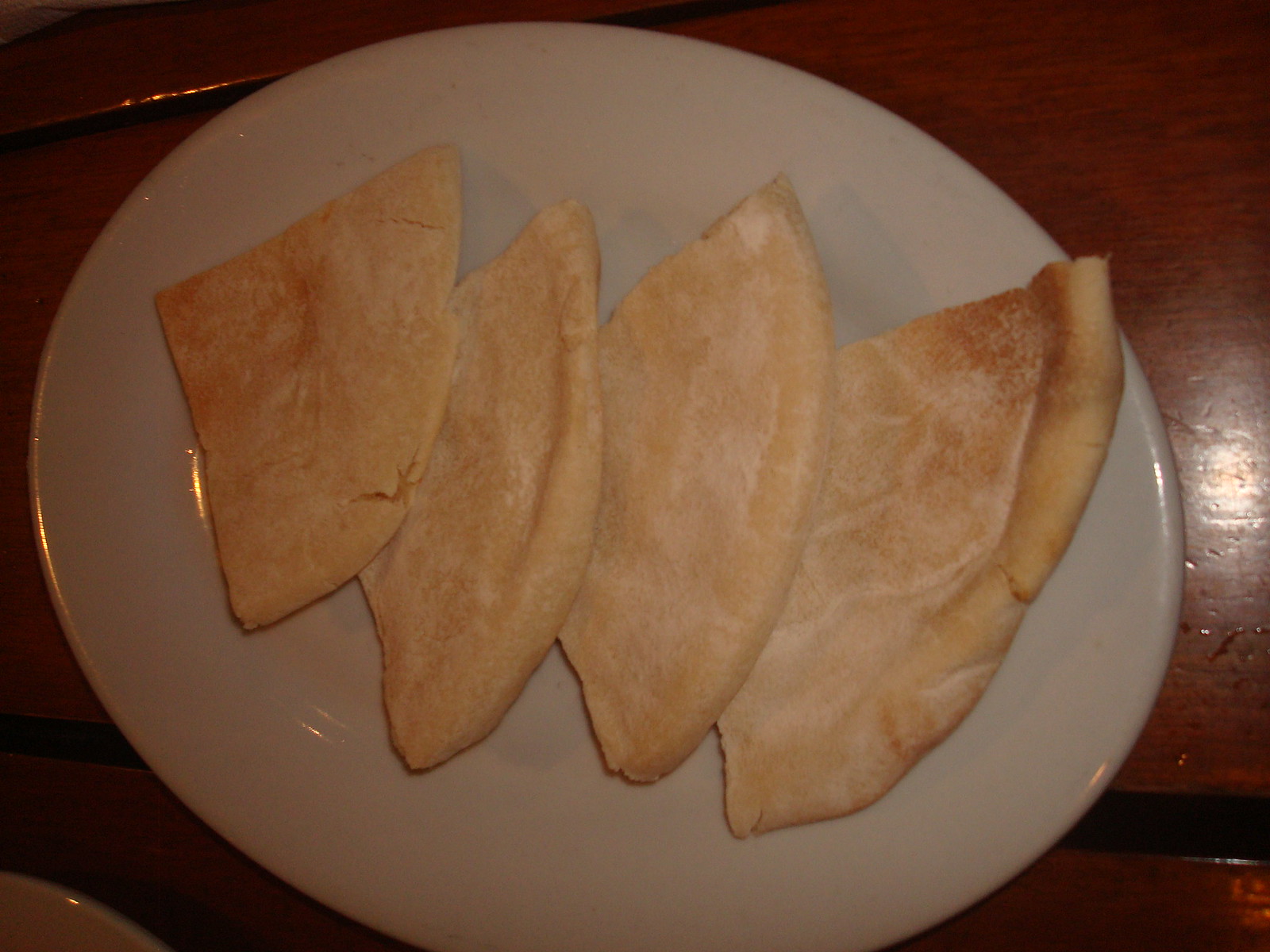This photograph is a top-down view of a low-quality snapshot featuring a white, oval-shaped plate, slightly cut off at the bottom. The central focus is four triangular slices of what appears to be a tortilla, flatbread, or pita, arranged in an overlapping pattern with their points facing the upper left. They are golden-brown with hints of light yellow and exhibit creases and textures that suggest they have been either baked or lightly fried, with some puffiness especially around the edges. A dusting of white flour and a sprinkling of brown sugar, likely cinnamon sugar, is visible on their surfaces. The plate rests on a sturdy brown wooden table that reflects the overhead lighting, highlighting the contrast between the dark red and bright tones of the table surface. The overall lighting is artificial, casting highlights and shadows that add depth to the image.